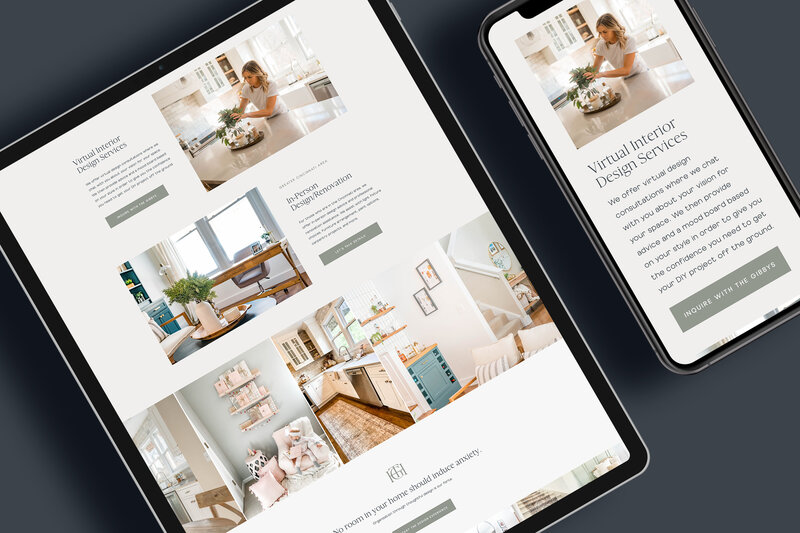The image is a left-to-right horizontal shot, and it appears to have been taken using a smartphone or computer. It looks like something that could be emailed to someone. The background is a flat, dark gray color without any texture or ombre effect, although some shadows create lighter and darker spots.

On the left side of the image, there's a tablet, and on the right side, there is a smartphone. Both devices display an advertisement for a virtual interior design service. The advertisement features a woman working in a modern white kitchen, and the text reads "Virtual Interior Design Services" in black. Below this text, there is a brief description of the service and a gray button to click for more information.

The advertisement also mentions "In-Person Design Renovation" and showcases a picture of a living room. Beneath this section, there is another blurb and a gray button for additional information. The bottom of the advert has more images that illustrate the services offered, accompanied by the tagline "No room in your home should induce anxiety." It also features the company's emblem and another gray button to click.

On the smartphone, the focus is on the woman in the kitchen with the accompanying text "Inquire with the Gibbys." The layout and information are similar, although condensed to fit the smaller screen.